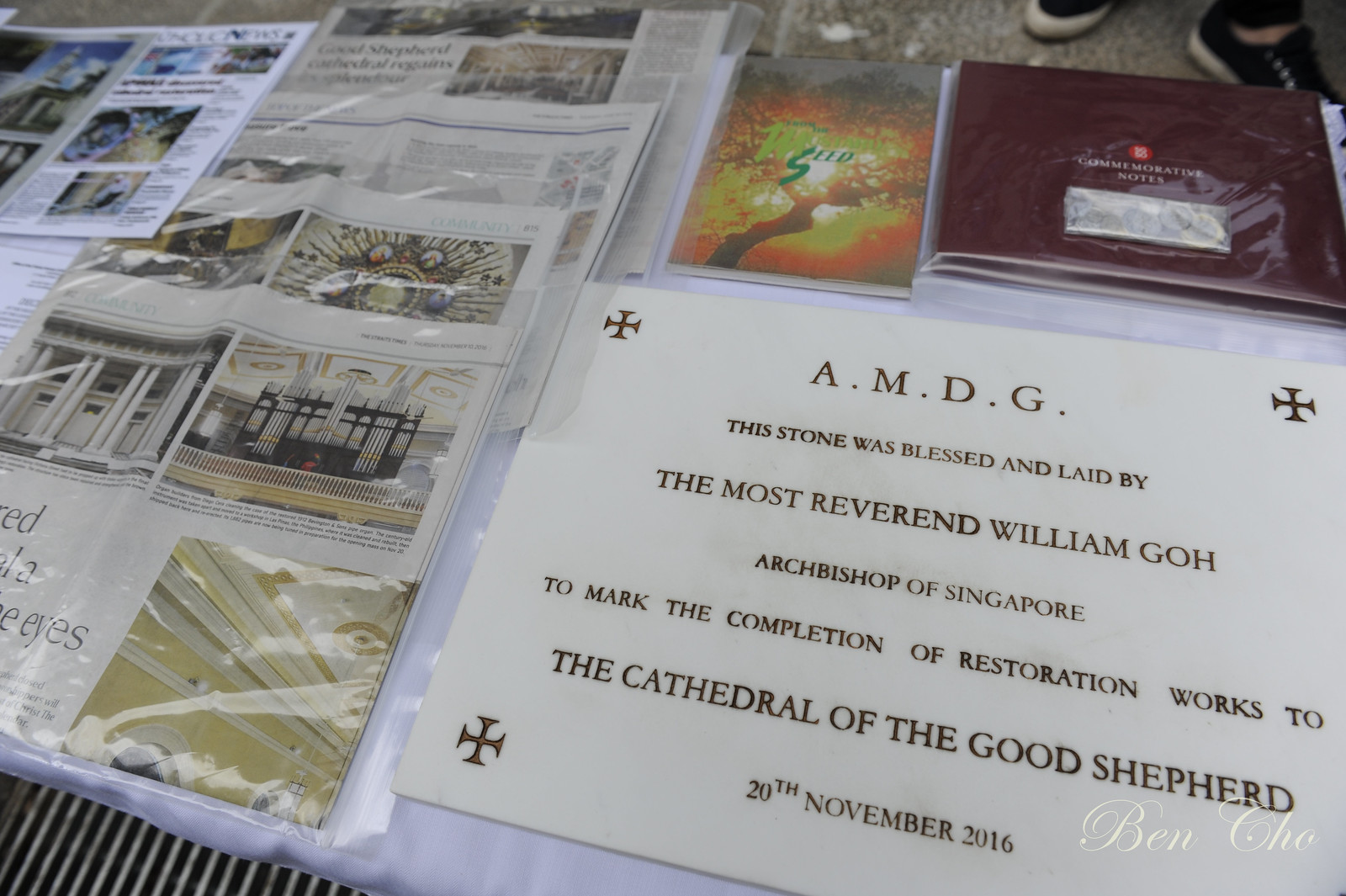The photograph captures a detailed and symbolic scene centered on a marble plaque laid flat on the ground. The plaque reads "A.M.D.G." at the top and features an inscription that states: "This stone was blessed and laid by the Most Reverend William Goh, Archbishop of Singapore, to mark the completion of restoration works to the Cathedral of the Good Shepherd, 20th November, 2016." The plaque has an ornate cross on each corner, emphasizing its religious significance. Surrounding the plaque, particularly to its left and above, are newspapers and books wrapped in clear plastic for protection. The newspapers likely discuss the restoration efforts of the cathedral, while one of the books appears to be commemorative notes. Also present are pictures of various stages of the cathedral’s restoration, further illustrating the historical importance of the event commemorated by the plaque.